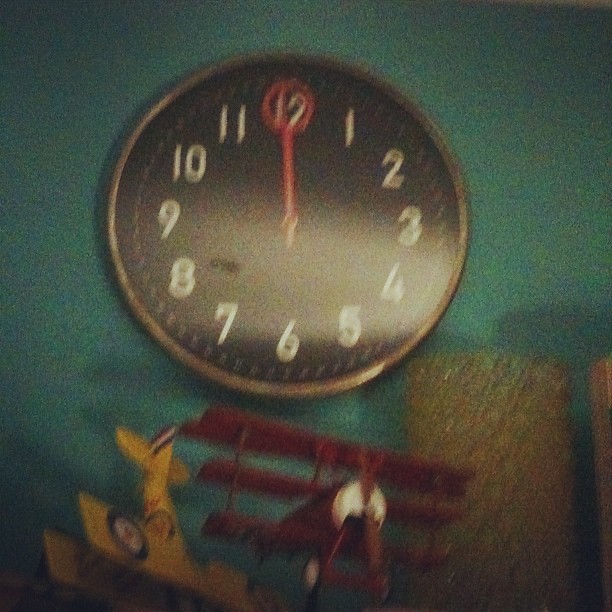A highly blurry and grainy photograph depicts a circular wall clock with a silver edge, mounted on a teal-colored wall. The clock features a black face with white traditional numbers and red hands, both pointing straight up to the twelve. Surrounding the clock are shadows that deepen towards the edges of the image. Below the clock, an old-style model airplane painted red faces toward the right corner of the photo, while a yellow model plane with blue target detailing is oriented downwards. To the right of the planes, partially obscured by shadows, a yellowish rectangle is visible. The overall low quality of the photo makes distinguishing details a challenge.